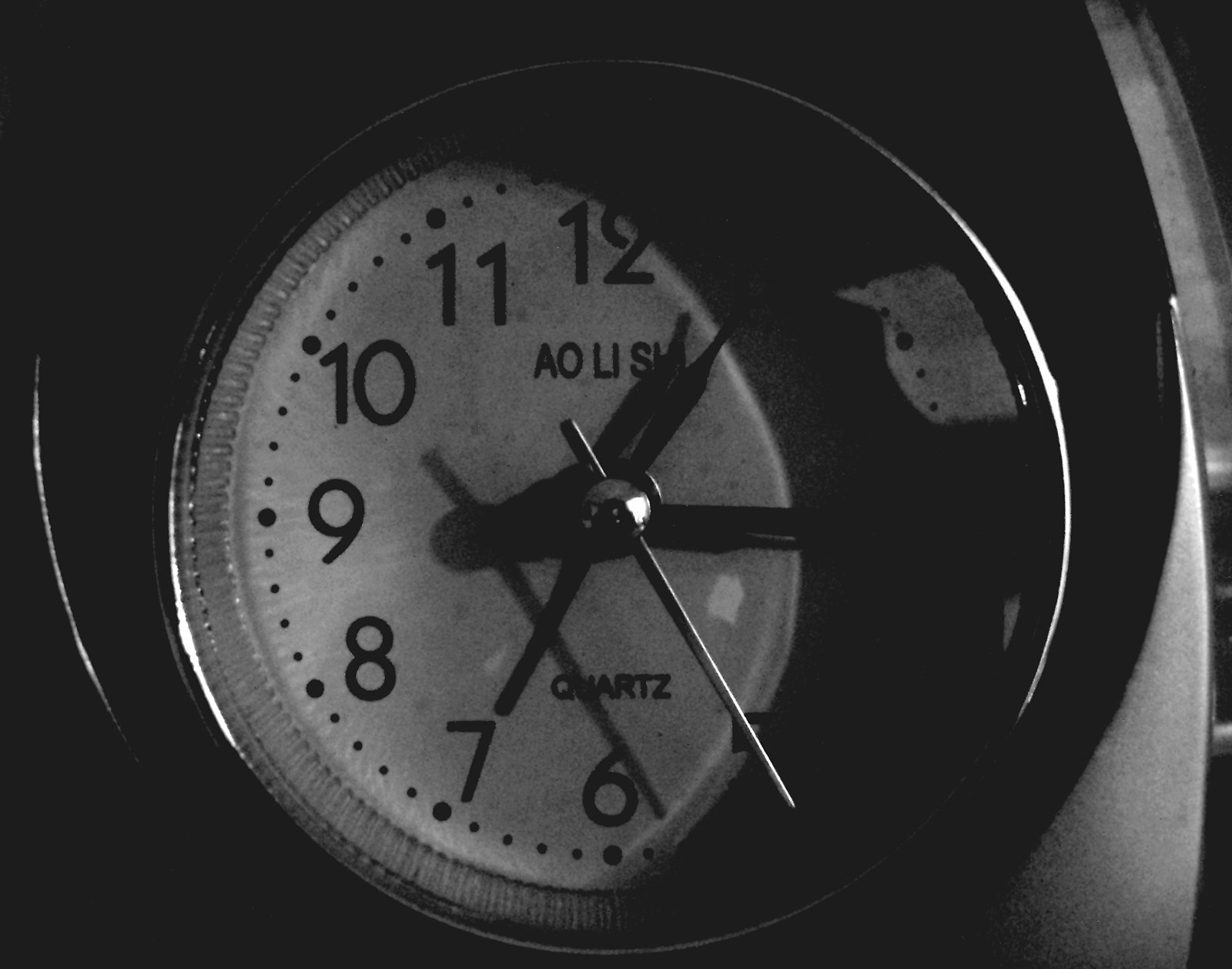This is a detailed black and white photograph featuring an up-close view of a clock positioned centrally in the frame. The clock is mostly enveloped in shadows, with only part of the left side clearly visible. The numbers 6 through 12 are discernible on this exposed side, and a faint hint of the number 5 is also noticeable. The clock's face transitions from a moon-shaped shadow covering the top and right side, creating a stark contrast between light and shadow. Three hands are visible: a short black hour hand, a long black minute hand, and an elongated silver second hand that connects to a raised central ball. These hands cast shadows on the clock face. At the top, just below the number 12, the letters "AOLISH" are inscribed, while "QUARTZ" appears prominently in capital black letters above the number 6. The perimeter of the clock features small black dots marking each minute, adding to the intricate detailing. The backdrop and surrounding areas of the image are predominantly dark, emphasizing the clock's silvery edge on the left and bottom sides. This nuanced lighting and composition lend an almost mysterious quality to the photograph.